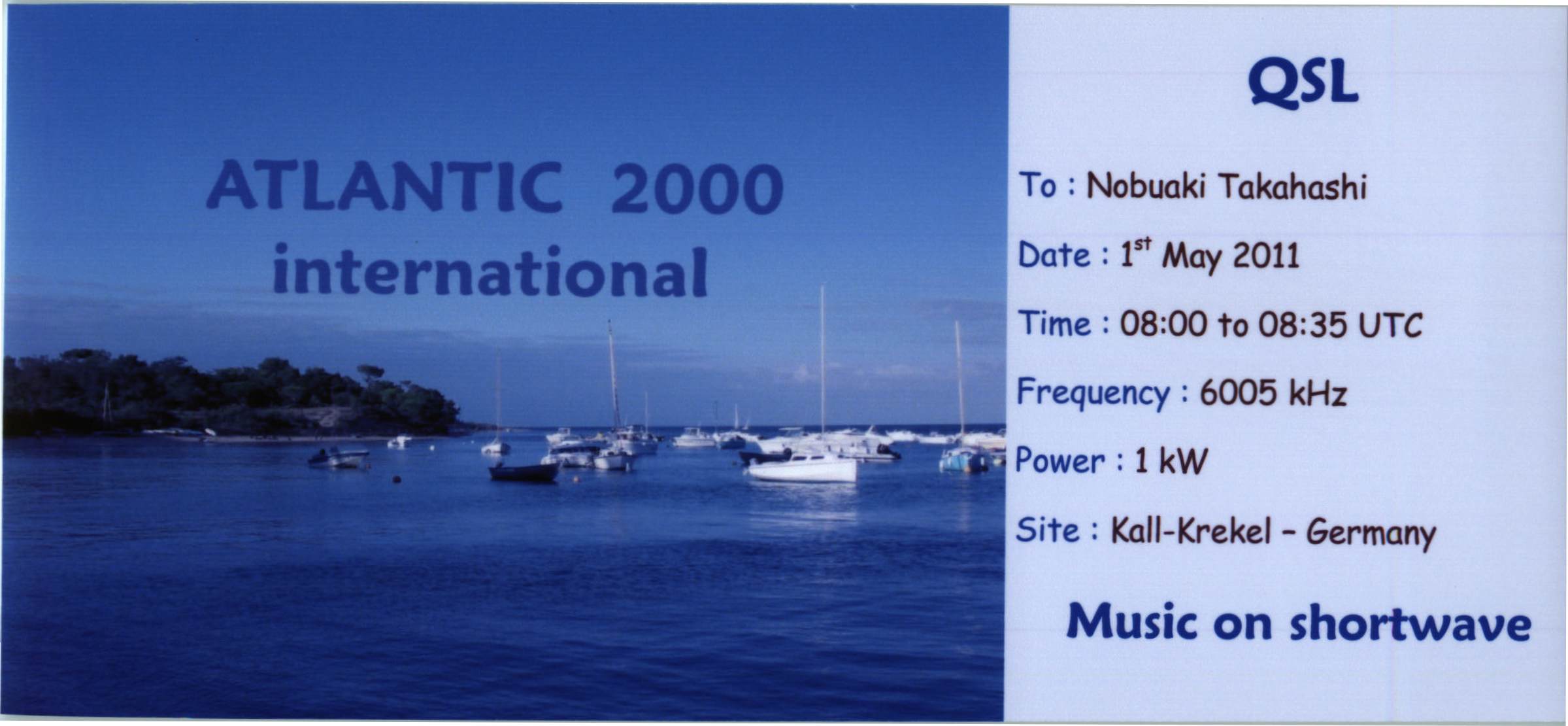The image features a rectangular postcard-like transmission receipt graphic. The card is divided vertically into two sections, with the left side occupying two-thirds of the space and the right side one-third. The left section showcases a vivid, deep blue image of a bay or marina with several docked sailboats, their sails down. A small island with trees is visible near the midline, and above that is a clear blue sky. Overlaying the image in bold blue text are the words "Atlantic 2000 International." 

The right section has a light blue background and contains detailed information about the transmission in dark blue and black text. At the top center, it reads "QSL" in dark navy blue bold print. The labeled information follows vertically on the left-hand side and includes:
- "To: Nobuaki Takahashi"
- "Date: 1st May 2011"
- "Time: 0800 to 0835 UTC"
- "Frequency: 6005 kHz"
- "Power: 1 kW"
- "Site: Cal-Carcle, Germany"

At the bottom in bold blue text, it states "Music on shortwave." The image is framed by a thin white border, and the overall color scheme includes shades of blue, green, white, and gray.